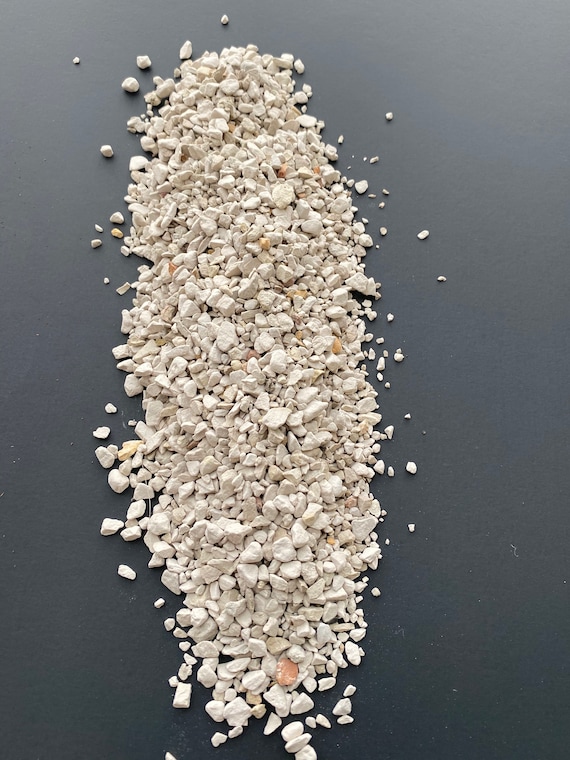The image features a vertical, elongated oval mound of small, tan-hued rocks and pebbles set against a dark gray background. The pile extends from the bottom to near the top of the vertically oriented photograph and is well-lit, showcasing each pebble in detail. Although predominantly tan, a few of the pebbles exhibit an orange hue, standing out against the lighter rocks. Scattered around the central mound, smaller pebbles break away from the main cluster. Each pebble closely resembles the size and shape of a pumpkin or sunflower seed. The background gradient is darker at the bottom, gradually lightening towards the top, creating a realistic photograph reminiscent of a textured surface such as a table.